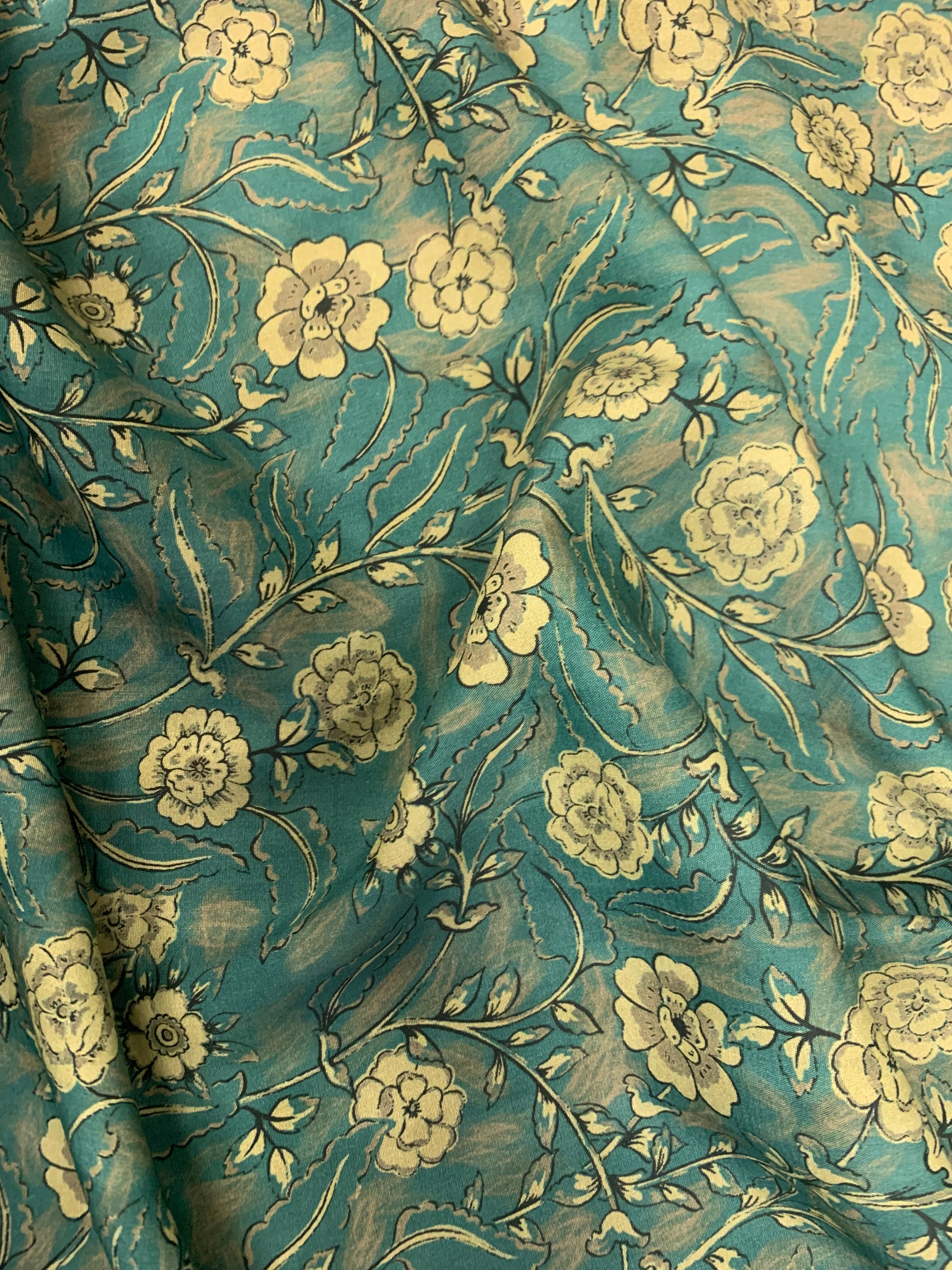The image is a detailed close-up of a decorated fabric or cloth with a richly textured pattern. The base color of the fabric is a dark greenish-blue, providing a vibrant background for the intricate design. The pattern showcases yellow or light gold vines and blossoms, with the vines adorned with small, delicate leaves. These yellow elements add striking contrast and intricacy to the cloth's surface. Besides the main blossoms and vines, there are additional light-colored designs interspersed throughout, contributing to the overall texture and depth of the fabric. Some of the leaves display darker tones, enhancing the sense of complexity in the design.

In the center of the image, a prominent fold in the fabric creates a dynamic visual effect, accompanied by a divot along the left corner, adding to the fabric's realistic and tactile quality. The cloth appears slightly rippled, perhaps gently billowing, suggesting movement or an aesthetically pleasing display, with no other objects or text in the background to distract from its intricate beauty. The overall impression is that of a meticulously crafted textile showcasing a harmonious blend of colors and patterns.